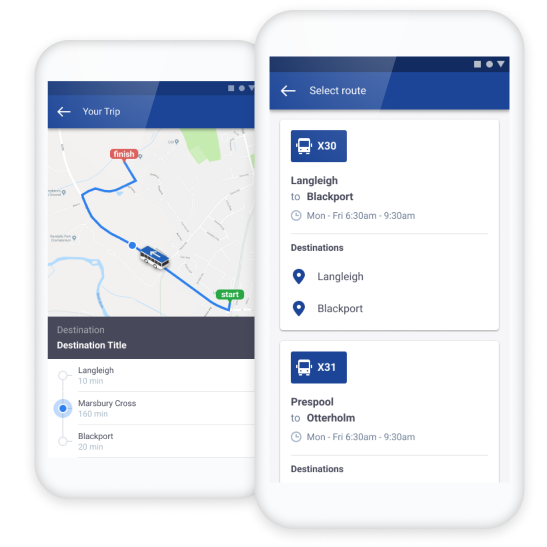A digital image displays two smartphone mock-ups, resembling iPhones but with simplified features. The left phone shows a navigation screen where the user is midway through a journey from Langley to Blackport. The trip duration is oddly segmented: from Langley, it indicates 10 minutes to an unnamed midpoint, followed by 160 minutes to another point, and finally 20 minutes to Blackport, adding up to an unclear total time.

The right phone screen reveals a detailed route selection interface, presenting three different route options for the same journey. Each route is marked with individual stops and varying travel times, allowing the user to choose their preferred path. The app appears to offer a comprehensive overview of different possible journeys, highlighting specific stops and durations.